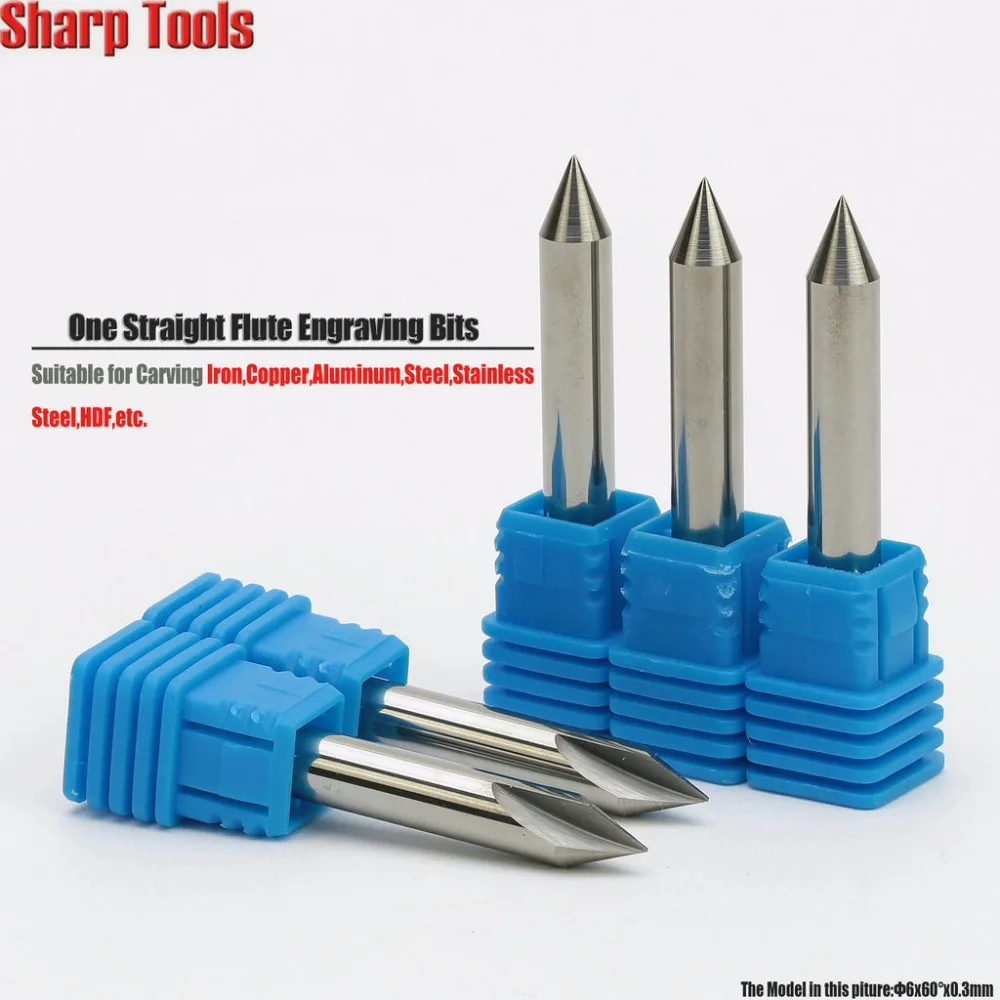This image features five sharp tools identified as straight flute engraving bits. These bits, constructed from metal and sporting a conical point, are nestled in blue plastic bases, which have a series of five stacked rectangular layers. In the setup, three of the bits stand upright, while the other two lie side by side in front of them, resembling Phillips screwdrivers with their jagged edges and pointed tips.

The image has a clean gray background, providing contrast to the vibrant blue bases and metallic bits. In the upper left corner, bold red text reads "Sharp tools," followed by black text below it that states "One straight flute engraving bits." This text is underlined and further supplemented by a description in gray text, "Suitable for carving iron, copper, aluminum, stainless steel, HDF, etc."

In the lower right corner, the model size is clearly indicated in dark black letters: "The model in this picture is 6 by 60 by 0.3 millimeters." The detailed description and the specific arrangement of the bits emphasize their precise engineering and versatile use in carving various materials.